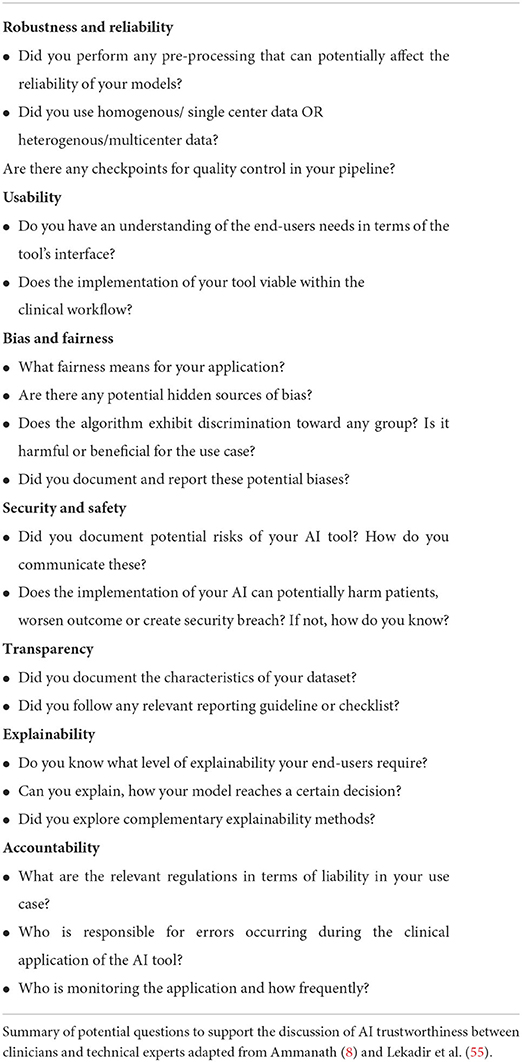### Capturing Comprehensive AI Implementation Considerations in Clinical Settings

**Image Description:** The image contains a detailed, bullet-pointed list of considerations for deploying AI tools, presented as black text on a white background. The list addresses several critical factors to ensure the robust, reliable, and ethical implementation of AI in clinical environments.

**Top to Bottom Breakdown:**

1. **Robustness and Reliability**
   - *Pre-processing Impacts:* Have you performed any pre-processing steps that could potentially affect the reliability of your AI models?
   - *Data Nature:* Did you use homogeneous (single-centered) data or heterogeneous (multi-centered) data?
   - *Quality Control:* Are there any checkpoints for quality control integrated into your pipeline?

2. **Usability**
   - *User Needs:* Do you have a clear understanding of the end user's requirements regarding the tool's interface?
   - *Workflow Integration:* Is the implementation of your tool viable within the existing clinical workflow?

3. **Bias and Fairness**
   - *Fairness Definition:* What does fairness mean in the context of your application?
   - *Bias Sources:* Are there any potential hidden sources of bias in your data or model?
   - *Discrimination:* Does the algorithm exhibit discrimination towards any group, and is this harmful or beneficial for the intended use case?
   - *Bias Documentation:* Have you documented and reported these potential biases?

4. **Security and Safety**
   - *Risk Documentation:* Have you documented potential risks associated with your AI tool, and how do you communicate these?
   - *Harm Potential:* Could the implementation of your AI tool potentially harm patients, worsen outcomes, or create security breaches? If not, how have you determined this?

5. **Transparency**
   - *Data Characteristics:* Did you document the characteristics of your dataset?
   - *Guideline Adherence:* Did you follow any relevant reporting guidelines or checklists?

6. **Explainability**
   - *User Requirements:* Do you know the level of explainability your end users require?
   - *Model Decisions:* Can you explain how your model reaches certain decisions?
   - *Complementary Methods:* Did you explore complementary explainability methods?

7. **Accountability**
   - *Regulations:* What are the relevant regulations regarding liability in your use case?
   - *Error Responsibility:* Who is responsible for errors that occur during the clinical application of the AI tool?
   - *Monitoring:* Who is monitoring the application, and how frequently are they doing so?

**Conclusion:** This comprehensive list underscores the importance of considering various aspects such as robustness, usability, fairness, security, transparency, explainability, and accountability when deploying AI tools in clinical settings to ensure their effective and ethical use.